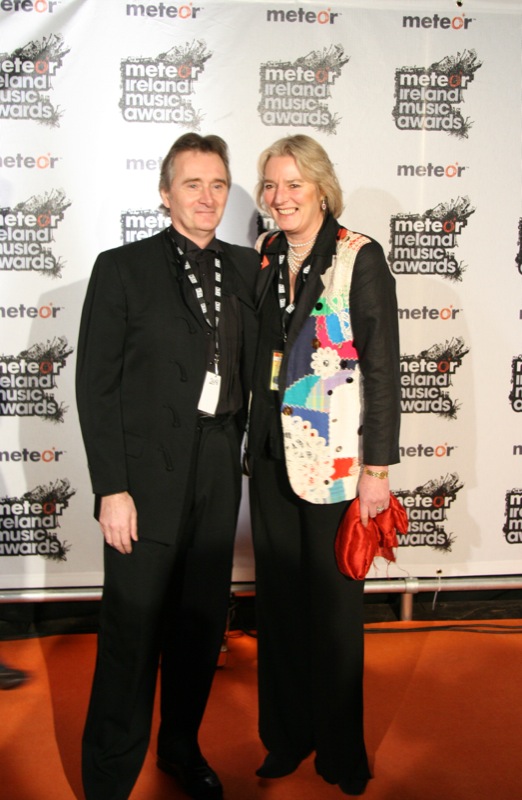In this detailed photograph, two middle-aged individuals, a man and a woman, are posed arm in arm on what appears to be a red carpet, set against a backdrop for the Meteor Ireland Music Awards. Both are likely musicians, given their attire and the event's context. The man, possibly in his late 50s or early 60s, has white skin and is dressed in a sophisticated all-black ensemble, including a black suit, a dark brown button-down shirt, and black shoes. He also wears a lanyard around his neck.

The woman beside him, also white-skinned and blonde with medium-length hair, exudes elegance in her colorful, patchwork vest jacket with black sleeves and a black lapel, complemented by a golden watch and a series of pearl necklaces. She holds an orange silk scarf in one hand and wears a black lanyard with a badge. Both are smiling warmly, their expressions directed at the camera, suggesting a posed moment for the paparazzi or event photographers. The backdrop reinforces the event's branding with repeated "Meteor Ireland Music Awards" logos, establishing the setting as a formal music award ceremony.